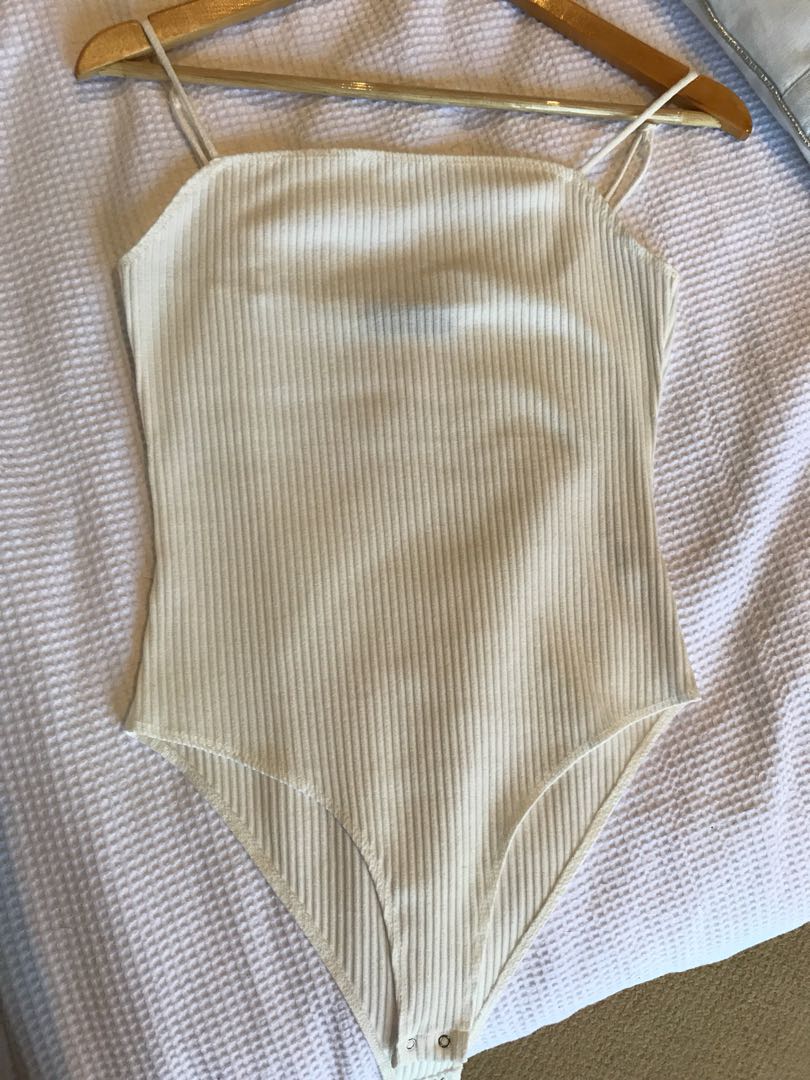This photograph features a cream-colored, ribbed fabric bodysuit with spaghetti straps and snap closures at the crotch. The one-piece garment is displayed on a wooden hanger, which is laid flat over a white, waffle-weave fabric that possibly covers a bed or couch. The overexposed lower right corner of the waffle-weave fabric suggests a casual, non-professional setting. The top portion of the hanger is cut off in the image, leaving only the bottom part visible. There is no text present in the photograph.